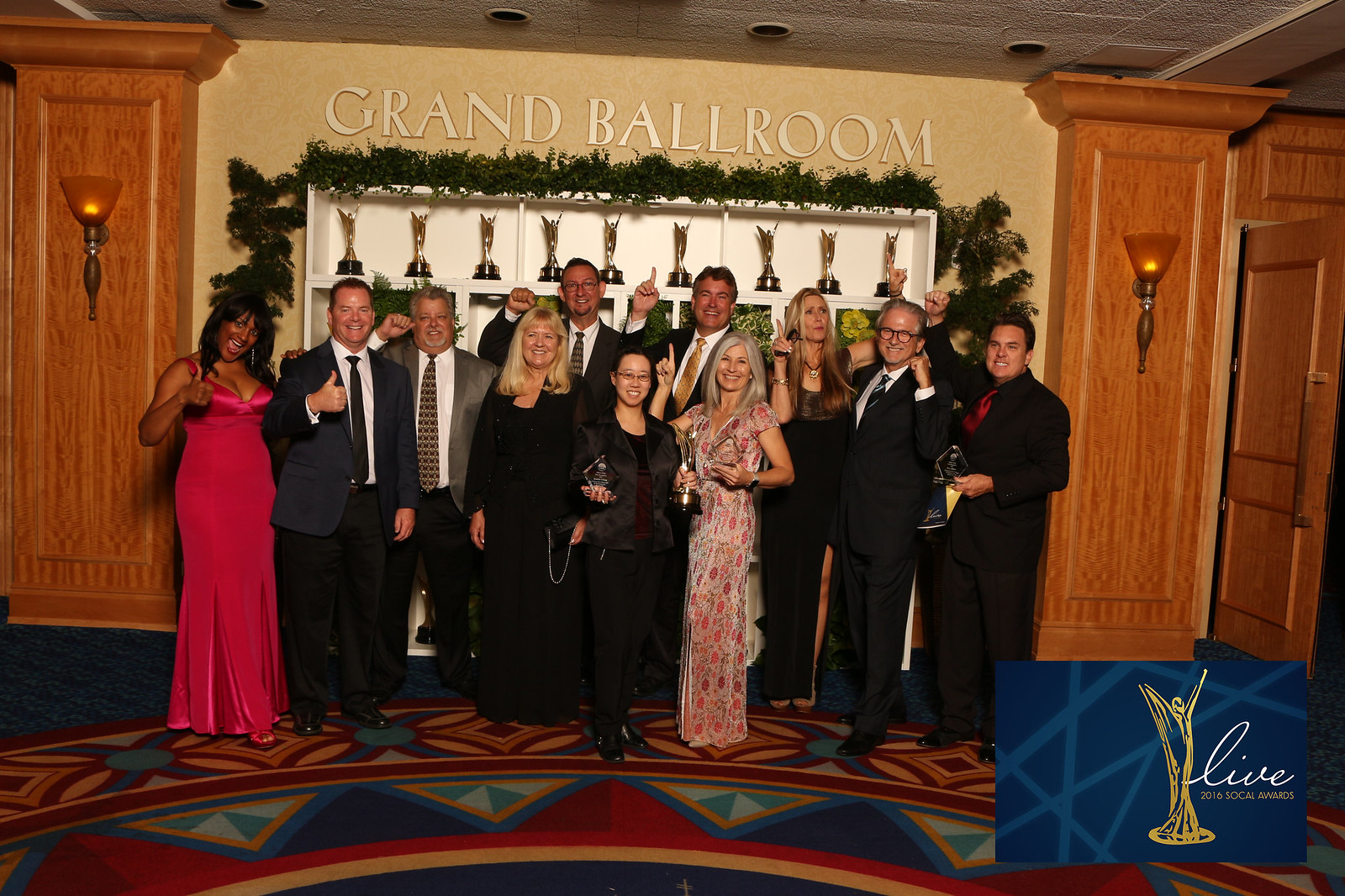This indoor photograph, set in a grand hotel, captures a formal group of eleven men and women posing in front of a trophy case in a ballroom hallway. The floor features a dark blue carpet with a colorful mosaic design incorporating triangles in red, blue, and yellow hues. Behind the group, there is a white shelf adorned with several identical trophies and greenery garlands wrapped around the top. Above the shelf, a sign reads "Grand Ballroom," and the surroundings include a stucco-like ceiling with recessed lighting. Flanking the group are two wooden pillars with wall sconces mounted on a yellowish wall. The men are dressed in suits and ties while the women wear long dresses, one notably in bright pink. Many are holding up a finger to signify being number one. In the bottom right corner of the photo, there's a blue pop-out image that features a trophy and the text "Live 2016 Social Awards."